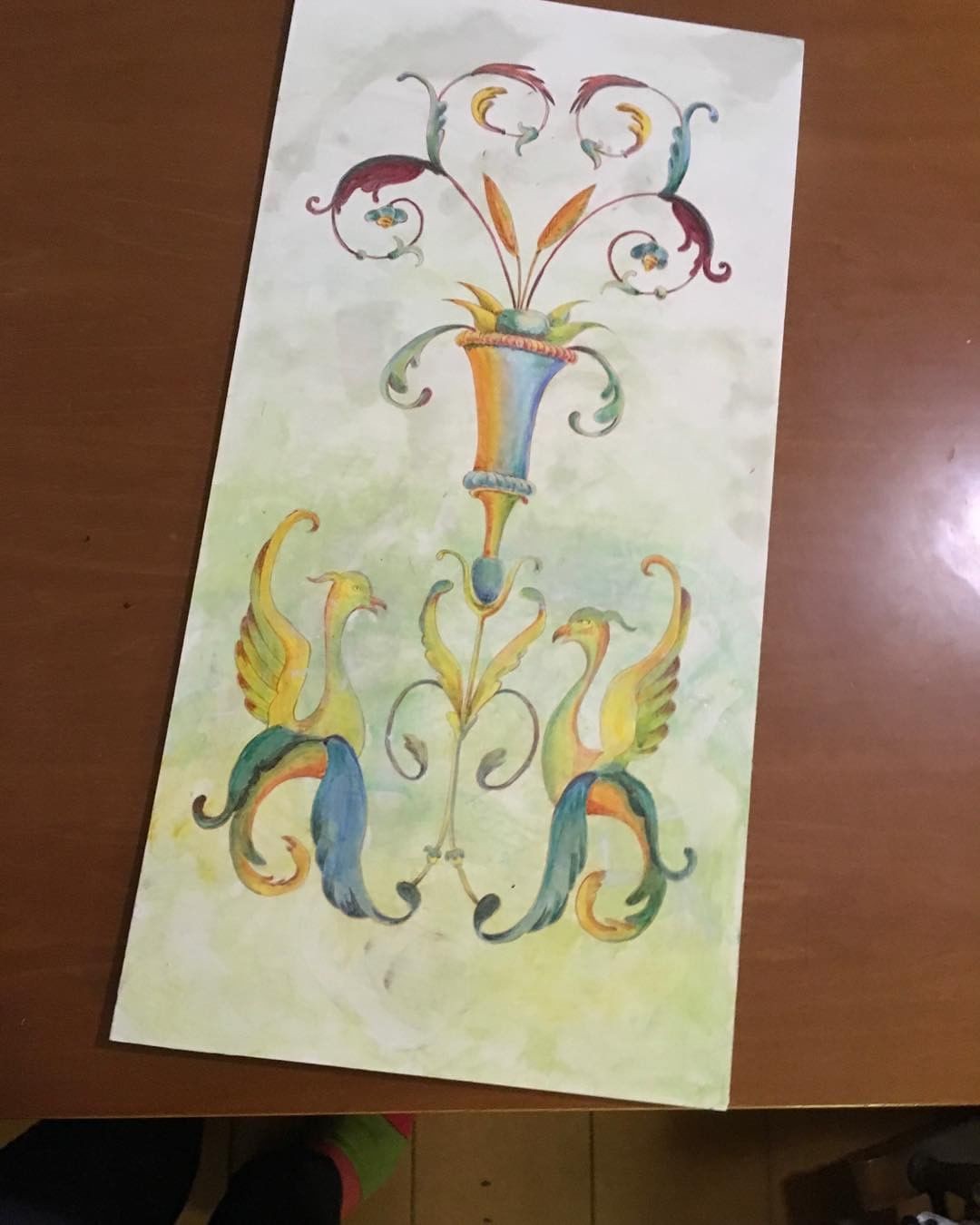The image showcases a vibrant painting, likely a watercolor, set against a wood grain wallpaper. The painting features an array of pastel colors including greens, blues, oranges, yellows, and browns. At the bottom of the painting, two birds, which are nearly identical and mirror images of each other, are portrayed with blue and green wings tinged with brown at the tips and some yellow hues. The birds, which resemble peacocks, have decorative feathers atop their heads.

Central to the composition is a multi-colored, blue and orange vase on a stand adorned with curlicue designs. Emerging from the vase are an assortment of feathers and floral elements, including maroon and reddish feathers, green foliage, and wheat sprigs. These elements are also mirror images, adding a sense of symmetry to the painting. Additionally, the ornate details include spirals and prominent orange-colored leaves.

The painting rests on what appears to be a brown wooden table. The overall backdrop includes various shades of yellow, green, white, and gray. The image further includes a glimpse of a tile floor and partial views of a person's feet, clad in green and pink socks, indicating that the photo is taken from above.